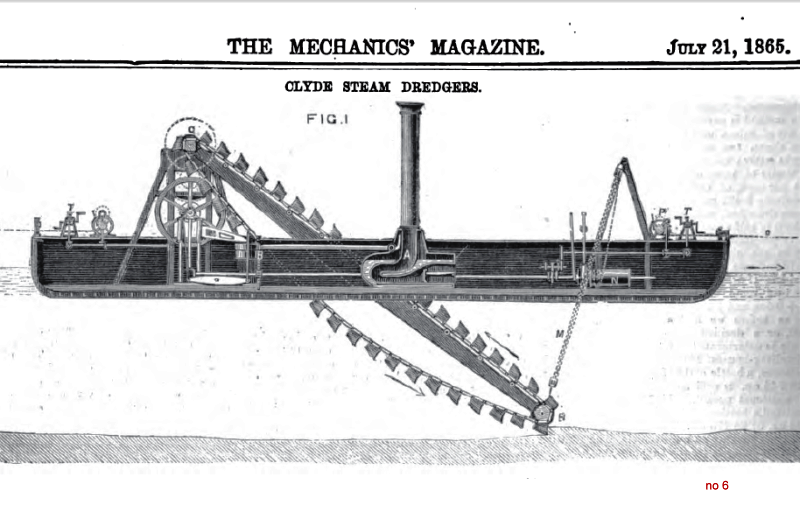This detailed black-and-white illustration from the July 21, 1865 issue of Mechanics Magazine showcases a Clyde Steam Dredger. The image, presented in landscape orientation, features finely detailed lines and is labeled at the top with "The Mechanics Magazine" in large capitalized letters. To the right, the date "July 21st, 1865" is clearly marked, separated by two horizontal black lines from the main illustration. Below, in slightly smaller lettering, it reads "Clyde Steam Dredgers," followed by a light-font inscription "Figure 1."

The central focus of the illustration is a long, narrow ship equipped with a prominent steam pipe rising from its center, indicative of steam power. The ship's function is accentuated by detailed mechanical elements; on the left side, an array of gears and a crank mechanism intricately connect to a conveyor belt. This conveyor belt descends beneath the water's surface, presumably to dredge sediment or soil, which is then transported to the back of the ship. Additionally, a mechanical arm on the right side of the steam pipe supports the belt's other end, ensuring efficient operation of the dredging process. The entire scene depicts the advanced engineering of its time, emphasizing the innovative design that allowed these dredgers to perform underwater excavation and sediment removal effectively.